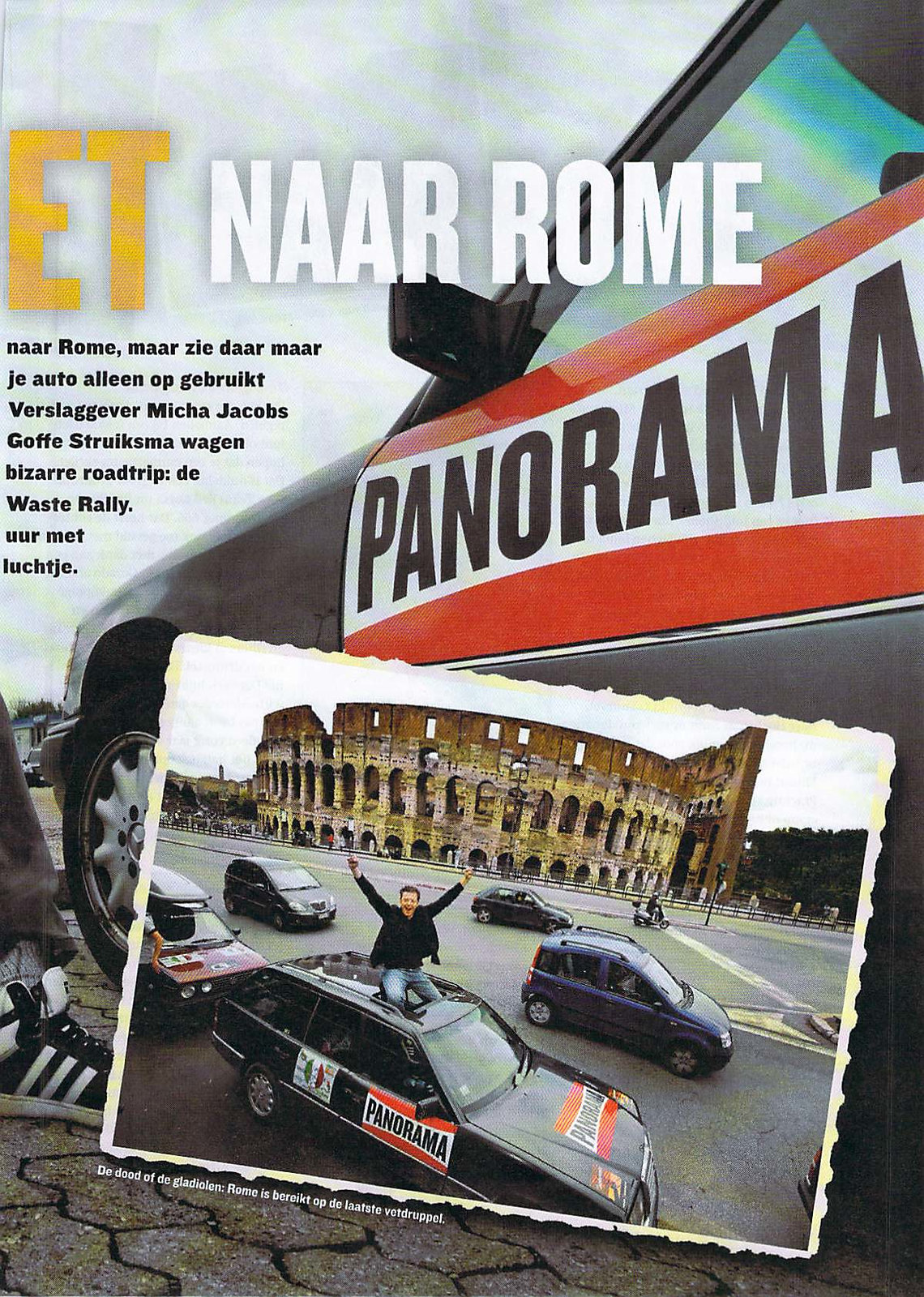This digital poster features a juxtaposition of two images with accompanying text. The background image showcases a car parked on a cobblestone street under a gray, cloudy sky. The car has "Panorama" written on the door in red, white, and black letters, with a red stripe along the top and bottom of the door. Beside the car, there is a visible leg wearing a black and white tennis shoe and black jeans.

Superimposed at the bottom of this background image is an inset picture, which appears to have torn edges. This inset displays a bustling road near a historical building similar to the Roman Colosseum. Among several vehicles, a blue and two black cars, the same "Panorama" car from the background is prominently featured. In this inset, a person is sitting on the car's roof, with his legs inside the vehicle through the sunroof. He is dressed in light-colored jeans and a black long-sleeve shirt or jacket, with arms raised in a V and a smiling expression, under the same cloudy sky.

The title of the poster is in bold yellow and white text at the top, reading "ET NAROM near Rome". Below this, smaller text in black, likely in different languages, lists names: "NAROM MARZI DARMAR J OTTO ALLEN OPP GABRIELT WERSLEY GOVER MECHA JACOBS GOFFE STRUELKSMA WEGEN BIZZA ROADTRIP T WEST RALLY URMET LACHCHE."